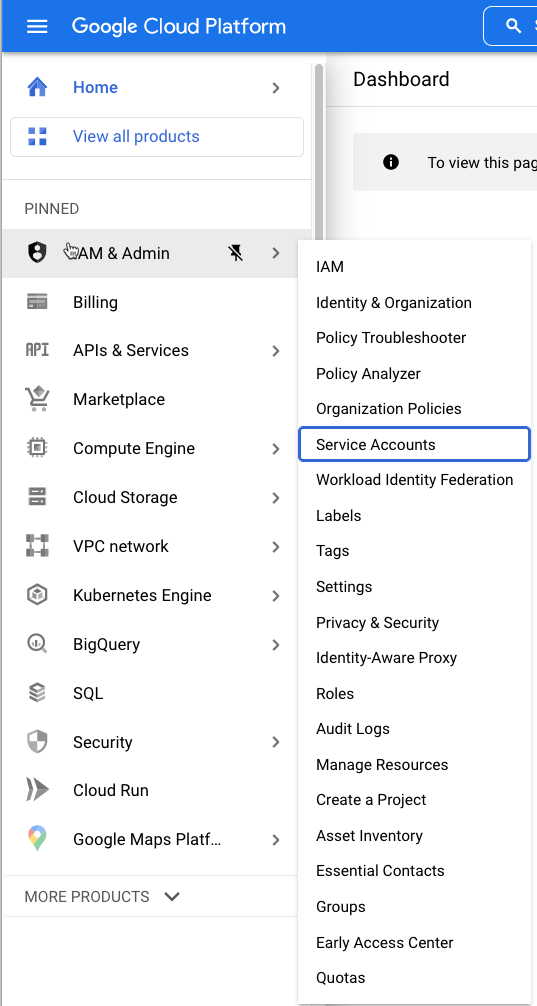This image is a cropped screenshot of the Google Cloud Platform web page. At the very top, there's a blue banner, within which the element on the far left is a hamburger menu icon represented by three horizontal lines. Following this, the text "Google Cloud Platform" is prominently displayed. On the far right of the screenshot, though partially cut off, is the search bar. The main background of the web page itself is white.

In the upper section of the main content area, there is a breadcrumb-like navigation path starting with the word "Home" accompanied by an arrow pointing to the right. Below this, the text "View All Products" is displayed. Down the left side, there is a sidebar titled "Pinned," listing items vertically with a scrollbar on the right, allowing further navigation through the list. In this "Pinned" section, the "GAM and admin" item is selected, revealing another vertical list underneath it. Within this nested list, "Service Accounts" is highlighted with a blue box.

To the right of this sidebar is a larger content area of the web page, which is mostly cut off in the screenshot. It has the word "Dashboard" displayed at the top. Additionally, there's a pop-up box with an information icon saying, "To view this page" with the rest of the message cut off. The cropped screenshot appears to be focused on showing the specific steps needed to navigate to "Service Accounts" as part of a task on the Google Cloud Platform.